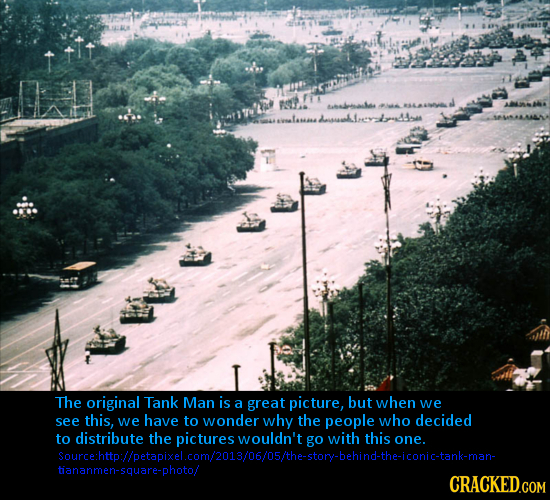This image captures the iconic scene from the Tiananmen Square protests, where a lone man stands defiantly in front of a long line of military tanks. The tanks, positioned in a single-file column, are moving down a tree-lined street with buildings and towers visible in the background. Surrounding the image is a layered caption: in a black box at the bottom, light blue text reads, "The original Tank Man is a great picture, but when we see this, we have to wonder why the people who decided to distribute the pictures wouldn't go with this one." Below this, darker blue text provides the source URL: "http://petapixel.com/2013/06/05/the-story-behind-the-iconic-tank-man-tiananmen-square-photo." In the lower right corner, "cracked.com" is displayed in yellow text.